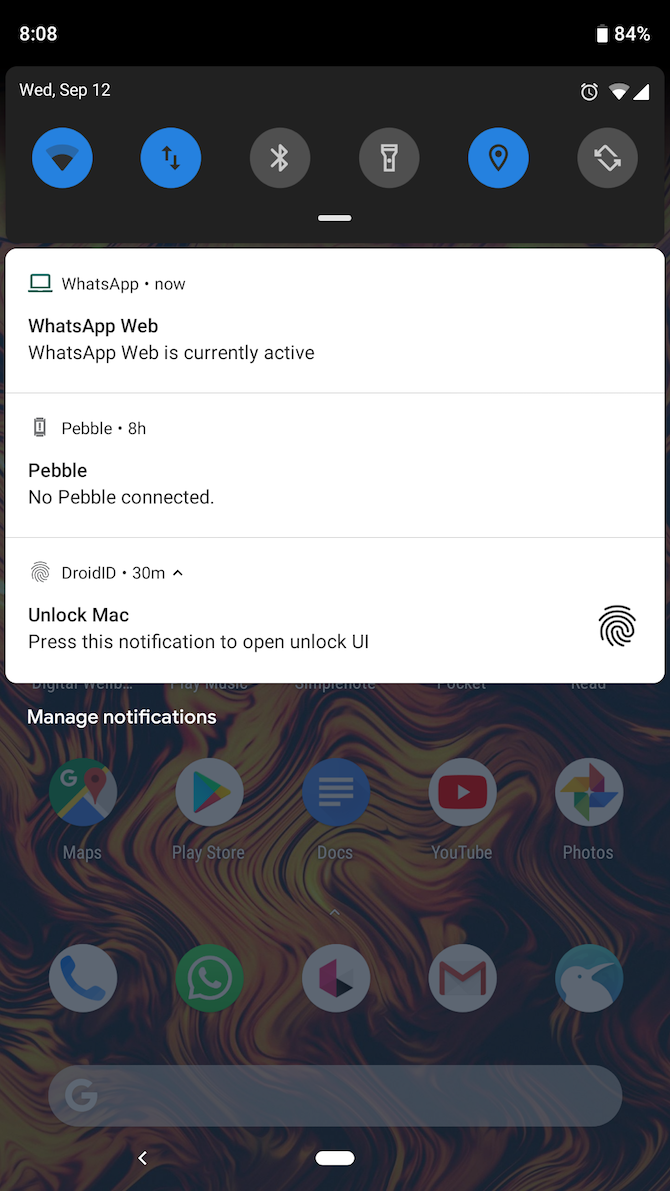The image showcases a smartphone screen with various details. The background is predominantly black with faint yellow and orange swirls barely visible beneath it.

At the top of the screen, in white text on the black background, it displays the time as "8:08" and the battery percentage as "84%". Below this information, also in black with white letters, it shows "Wednesday, September 12th".

Further down, there are six circles each containing different symbols. Below these circles, a notification banner appears:
- The first notification states: "WhatsApp Web is currently active".
- The second notification reads: "Pebble: 8 hours. No Pebble connected".
- The third notification indicates: "Droid ID: 30 minutes. Press this notification to unlock UI", and includes a fingerprint icon.

At the bottom of the screen, the text "Manage Notifications" is displayed. Below this text, there are two rows of grayed-out symbols, each row consisting of five icons, resembling telephone symbols.